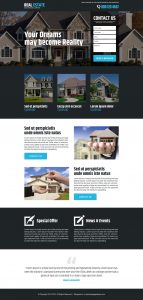In the image, a dreamlike scene is depicted where aspirations of homeownership are brought to life. A quaint two-story house stands in the background, surrounded by sporadic trees and patches of well-kept lawns. Despite the overall low quality and degradation of the image, the house's colors—primarily white, blue, and brown—remain discernible. In the forefront, a symbolic exchange of house keys takes place, signifying the completion of a home purchase or transfer. Along the bottom of the image, there are notifications, news messages, and upcoming events, although their specifics are too blurred to be legible. This visual composition suggests the realization of a dream and the beginning of a new chapter in a welcoming neighborhood. Contact us for more information and to make this dream a reality.